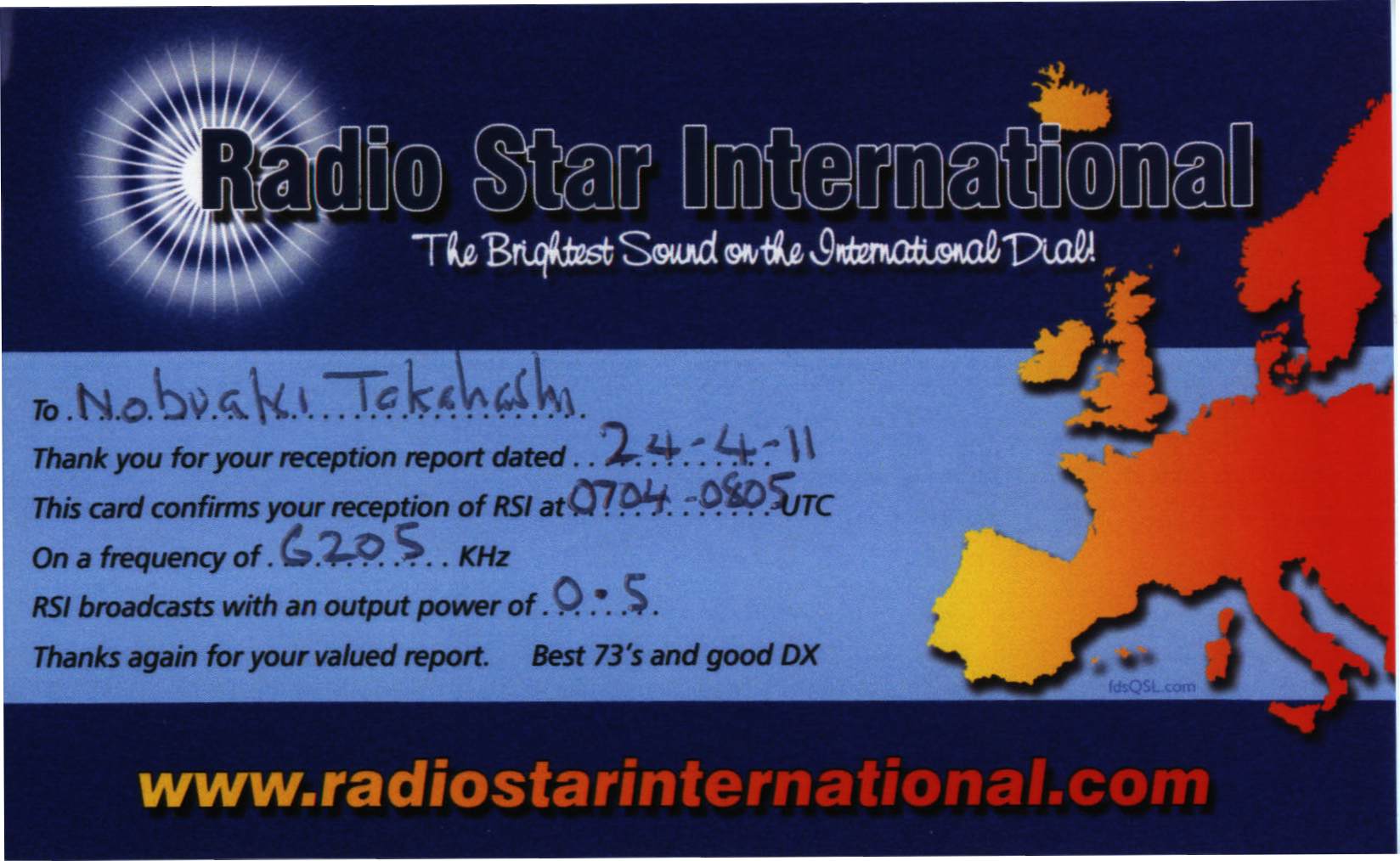The image depicts a slide with a dark blue background, prominently featuring the text "Radio Star International" at the top, overlaid with a blue and white sunburst design. The words "Radio Star International" are written in black font, making them slightly challenging to read against the dark background. Below this header, a white byline declares, "The brightest sound on the international dial," which stands out clearly. On the right side of the slide, there is a map in shades of orange and yellow displaying part of Europe, particularly everything west of Italy. The slide also contains a handwritten note addressed to Nobuaki Takahashi, thanking them for their reception report dated 24-4-11. It confirms the reception of RSI at 07040805UTC on a frequency of 6205 kHz, with an output power of 0.5. The closing note thanks again and wishes "best 73s and good DX," followed by the website www.radiostarinternational.com.